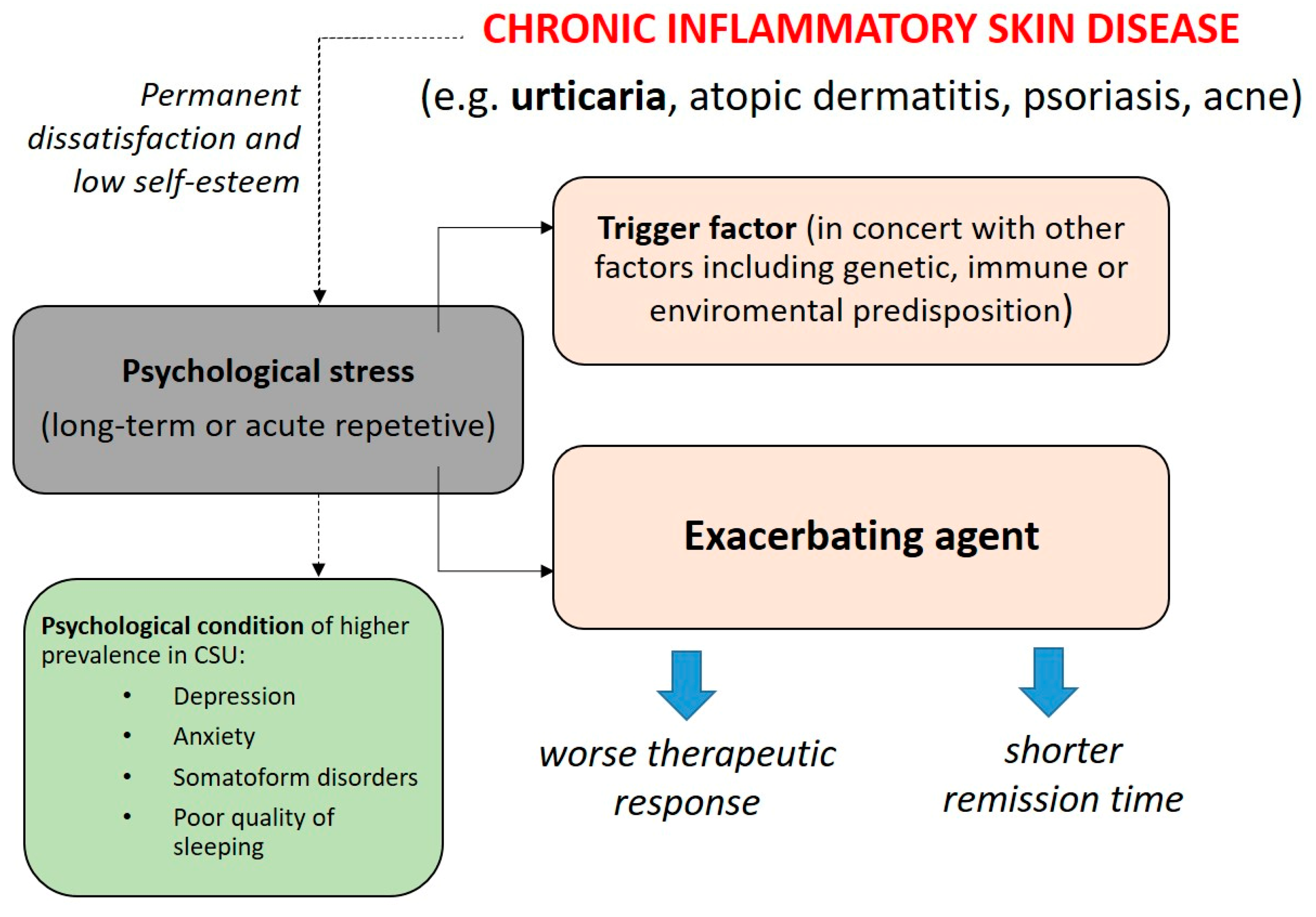In this detailed flowchart on chronic inflammatory skin disease, the title at the top is in bold red capital letters. Below this title, there is a dotted line leading down to a grey box labeled "psychological stress," with parenthetical text indicating both long-term and acute repetitive stress. Adjacent to this, on the left side, are black dotted lines that point to descriptions involving permanent dissatisfaction and low self-esteem.

Progressing down from "psychological stress," we encounter a blue box containing text about psychological conditions with higher prevalence in CSU, which include depression, anxiety, somatoform disorders, and poor sleep quality. Arrows extend from the "psychological stress" box: upwards to a white-pink box labeled "trigger factor," noting contributions from genetic, immune, or environmental predisposition; and downwards to a light pink box labeled "exacerbating agent." Below the "exacerbating agent" box, two thick blue arrows point further down to indicate negative outcomes: "worse therapeutic response" and "shorter remission time." Additionally, text beneath the main title clarifies examples of conditions, specifying urticaria, atopic dermatitis, psoriasis, and acne.